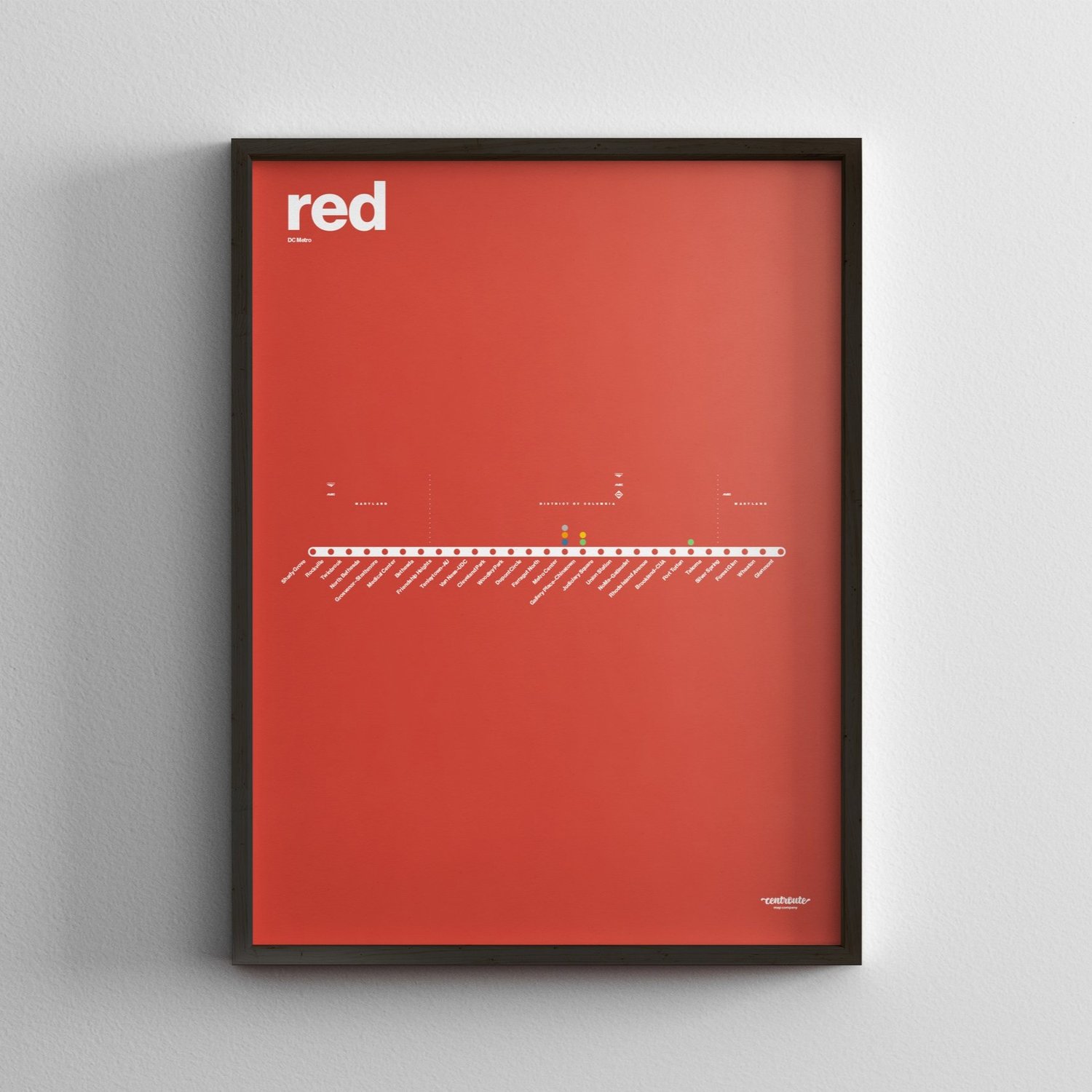The photograph depicts a black-bordered photo frame mounted on a light grey wall. Inside the frame is a vibrant red poster. At the top left corner of the poster, the word "red" is written in white lowercase letters. Running horizontally across the middle of the poster is a white line adorned with red and colorful dots above it, as well as smaller red dots on the line itself. Below this line, there is some text written in very small letters, which are difficult to read. Additionally, the bottom right corner of the poster contains more white text, also small and blurry. The poster is brightly lit, benefiting from the abundance of natural light, making the vivid colors and design details stand out sharply against the light grey wall.